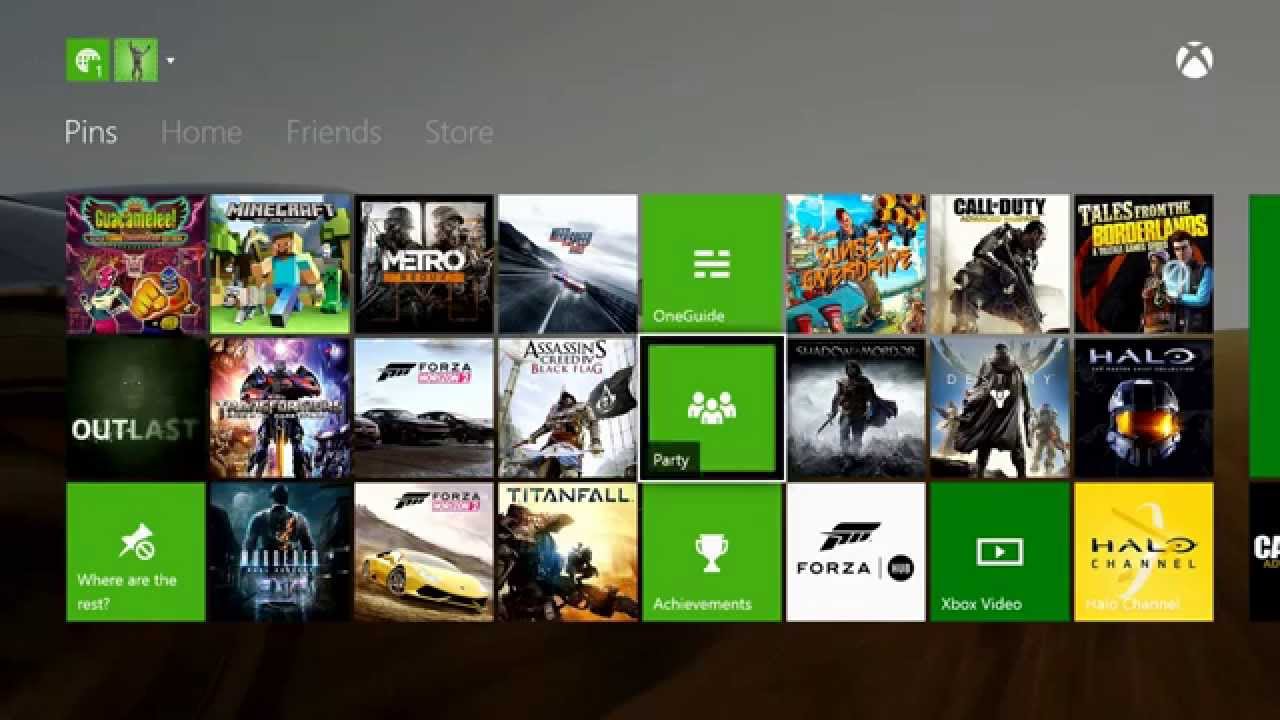This image showcases a video game interface loaded with diverse game selections. In the upper left corner, there are two prominent green squares. The first square contains the number "1," while the second square features an icon of a person with their arms raised above their head. To the left, the word "PENS" is displayed in bold white letters.

To the right of this section, the main menu categories: Home, Friends, and Store are clearly labeled. Dominating the upper right corner is the recognizable Xbox symbol, which is a white circle encasing a stylized "X."

The games are organized into three rows, each illustrating distinct game titles. The first row highlights Minecraft with its iconic blocky characters, Metro, a green square labeled One Guide in the center, an image of a soldier wielding a gun for Call of Duty, and Tales from the Borderlands.

In the second row, we have the horror game Outlast, featuring an eerie creature with bright white eyes, Transformers depicted with a colossal robot, Forza with a sleek car image, Assassin's Creed Battle Flag with a green square marked party, and finally, Halo.

The last row, in the bottom left corner, has a green box that reads "Where Are the Rest?" followed by more game selections, including Titanfall, Forza, and Halo Channel, which is uniquely highlighted within a yellow square.

Each element within this image collectively creates a vibrant and organized display of a gamer's paradise.